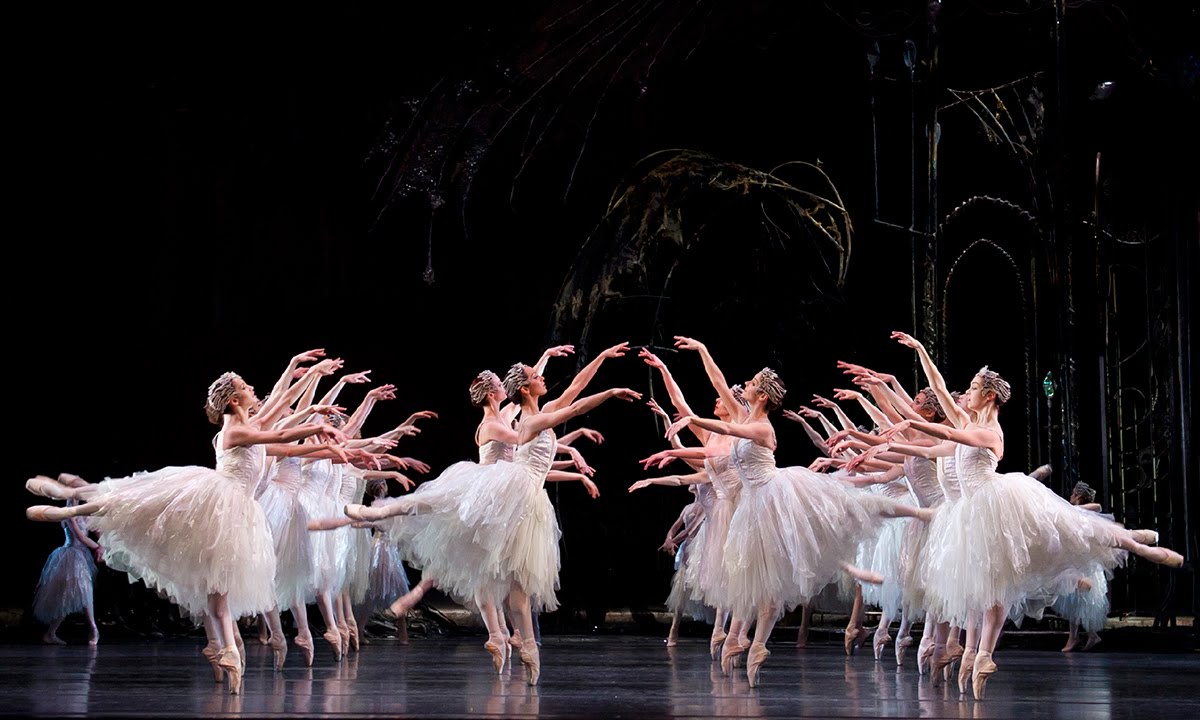The photograph captures a striking scene of a ballet performance on a dark stage. Approximately thirty ballerinas are arranged in four rows—two rows on the left and two on the right—facing each other. Each dancer is balanced gracefully on the tiptoe of one foot, with the other leg extended straight behind them in an elegant arch. They all wear identical white dresses adorned with layers of puffy, lacy, semi-transparent material at the bottom, complemented by white net tiaras that drape over their heads.

Their arms are positioned methodically: one arm extends straight in front with the hand loosely hanging, while the other arm is raised and pointing forward, also with a relaxed hand. The dancers in the centermost rows on the left and right are almost touching hands, creating a sense of symmetry and cohesion in their formation. In the backdrop, faintly visible props suggestive of archways of lights and bush-like branches on pillars add a hint of ambiance without detracting from the dancers' ethereal presence.